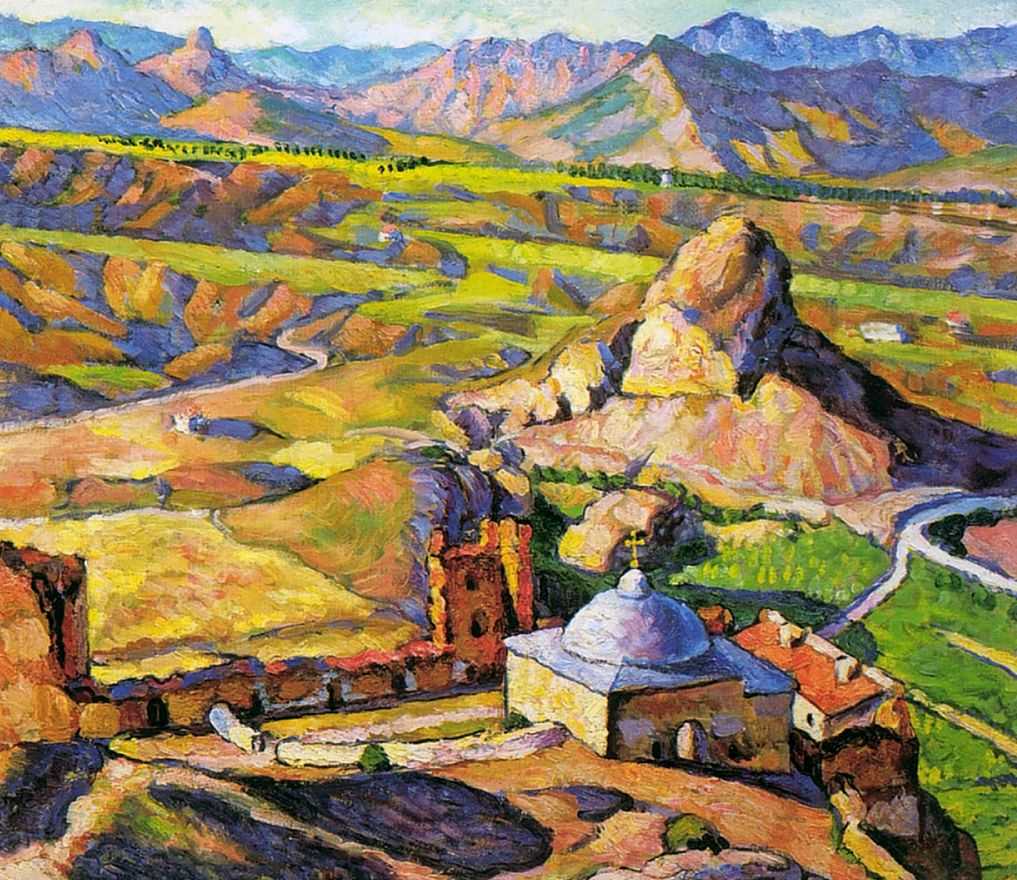The painting depicts a verdant village nestled in a valley characterized by a rich palette of pastel colors including orange, green, red, yellow, and pale hues. At the forefront stands a distinctive church with a circular dome topped by a gold cross. Adjacent to the church, there's a red-roofed building, possibly a home with two chimneys, and a large, castle-like structure made of red brick. A prominent rock pile and some ruins can be seen just beyond the church. Further into the valley, green cliffs slope down to a body of blue water, suggestive of a lake, lagoon, or river, bordered by a forest of trees. In the far distance, majestic mountains rise high into a partially cloudy but blue sky, highlighted with shades of blue, purple, and light green. The entire scene is imbued with a lush and pastoral charm.